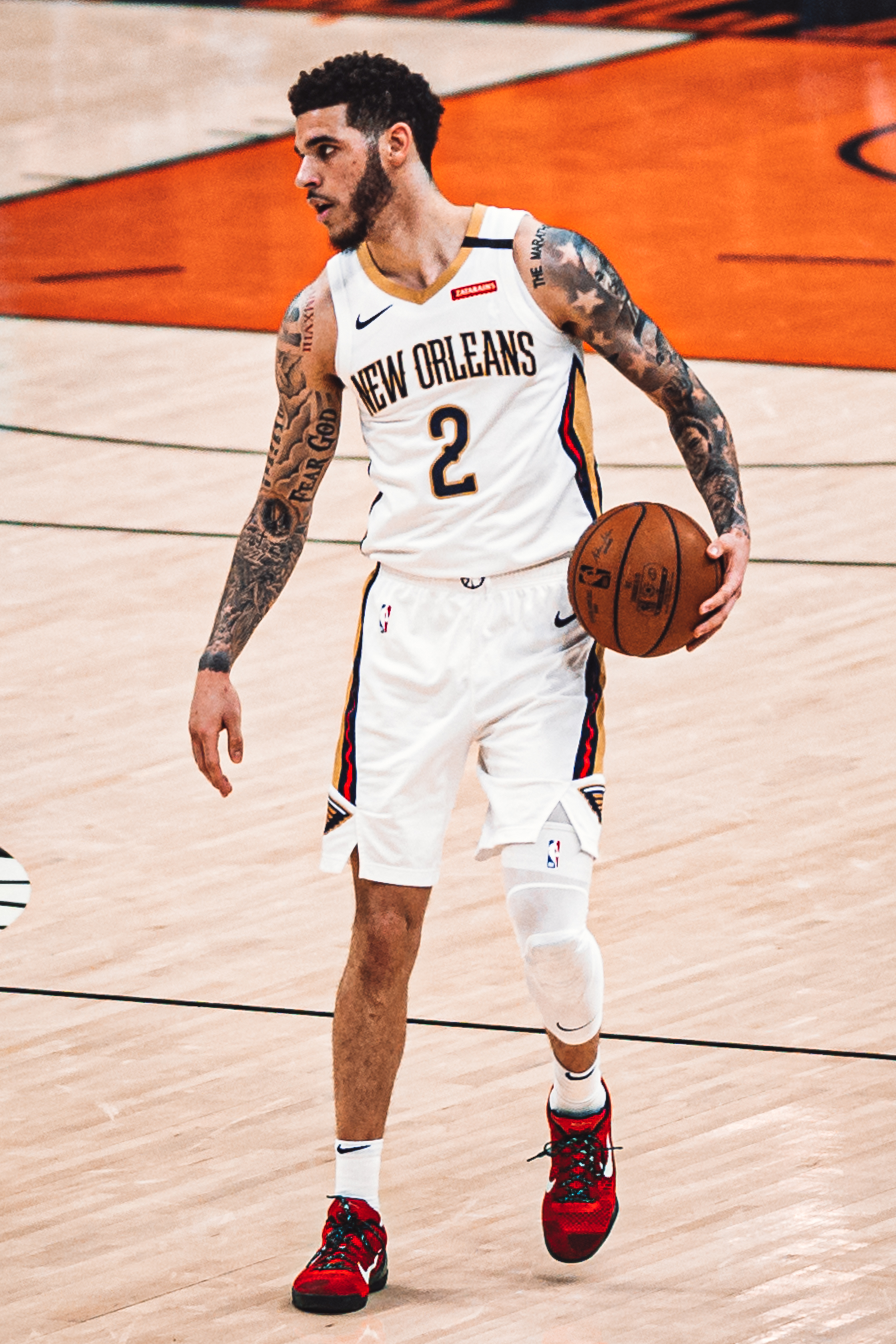In the center of this image, a basketball player stands prominently on a smooth hardwood basketball court, identifiable by the painted lines. The player, wearing a full uniform that reads "New Orleans" with the number two emblazoned on the front, is adorned in a white jersey featuring gold and reddish-brown stripes down the side. His heavily tattooed arms, covered from shoulder to wrist in detailed sleeve tattoos, are clearly visible. The player has dark, curly hair, a mustache, and a full beard. He is wearing predominantly red Nike shoes with black details and white socks, along with a noticeable knee brace on his left leg. Holding an orange basketball against his hip with one hand, he appears to be gazing off to the side, with his left foot slightly lifted off the ground. The setting appears to be an indoor basketball court with tan and orange hues, further emphasizing the athletic context of this scene.